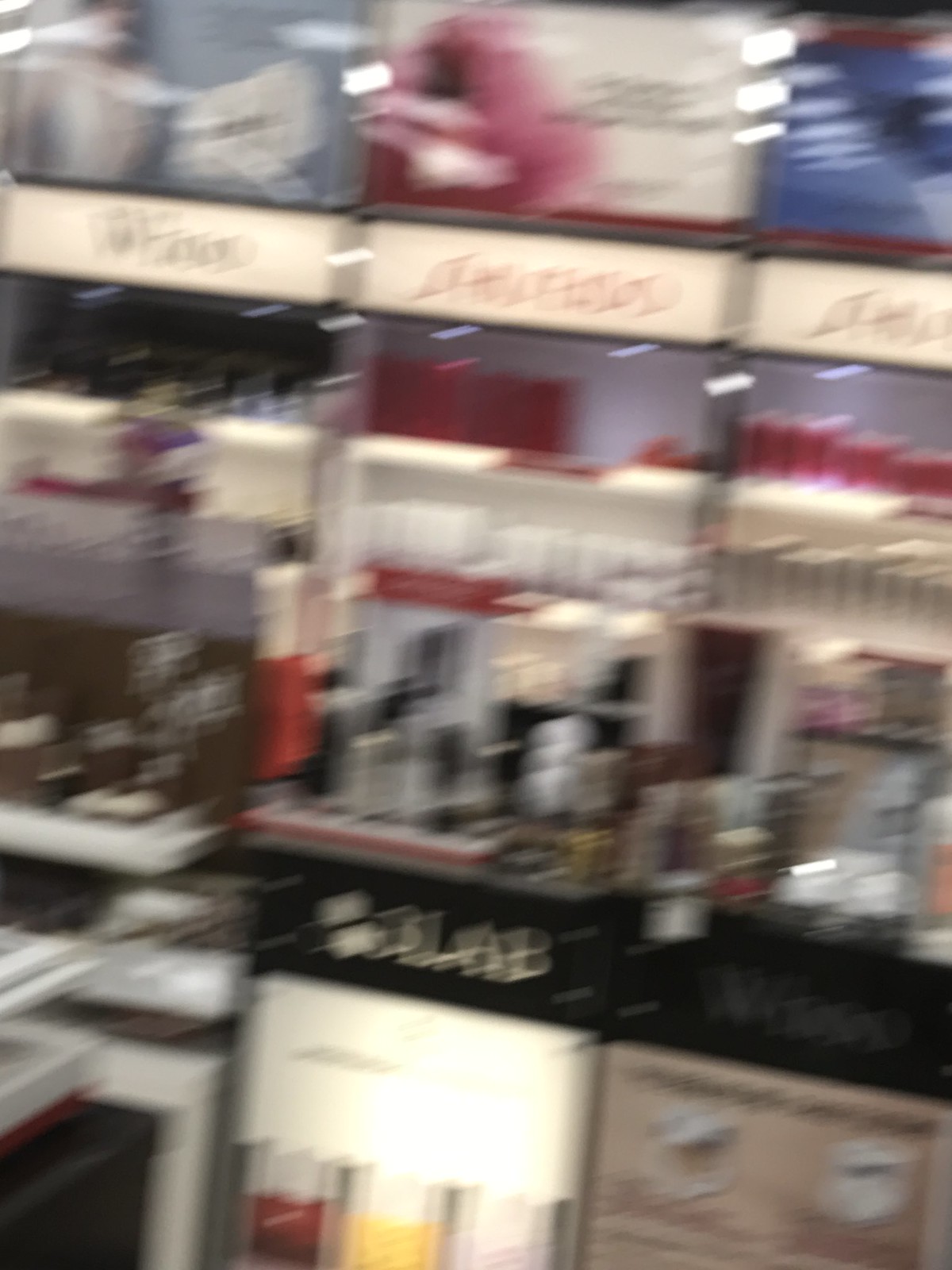A slightly angled, out-of-focus image capturing an extensive makeup counter inside a store. The wall of products displays various merchandise, though the specific names are not discernible due to the blurriness. Three signs are positioned at the top of the photo, with the center one clearly reading "Shiseido" in red. The left sign appears to spell out a brand name similar to Valentino, but with fewer letters, while the details of the right sign remain indistinct. The bottom right section of the photo features posters displaying different products. Shelves in the center of the image are stocked with a wide array of makeup products, enhancing the counter's display.